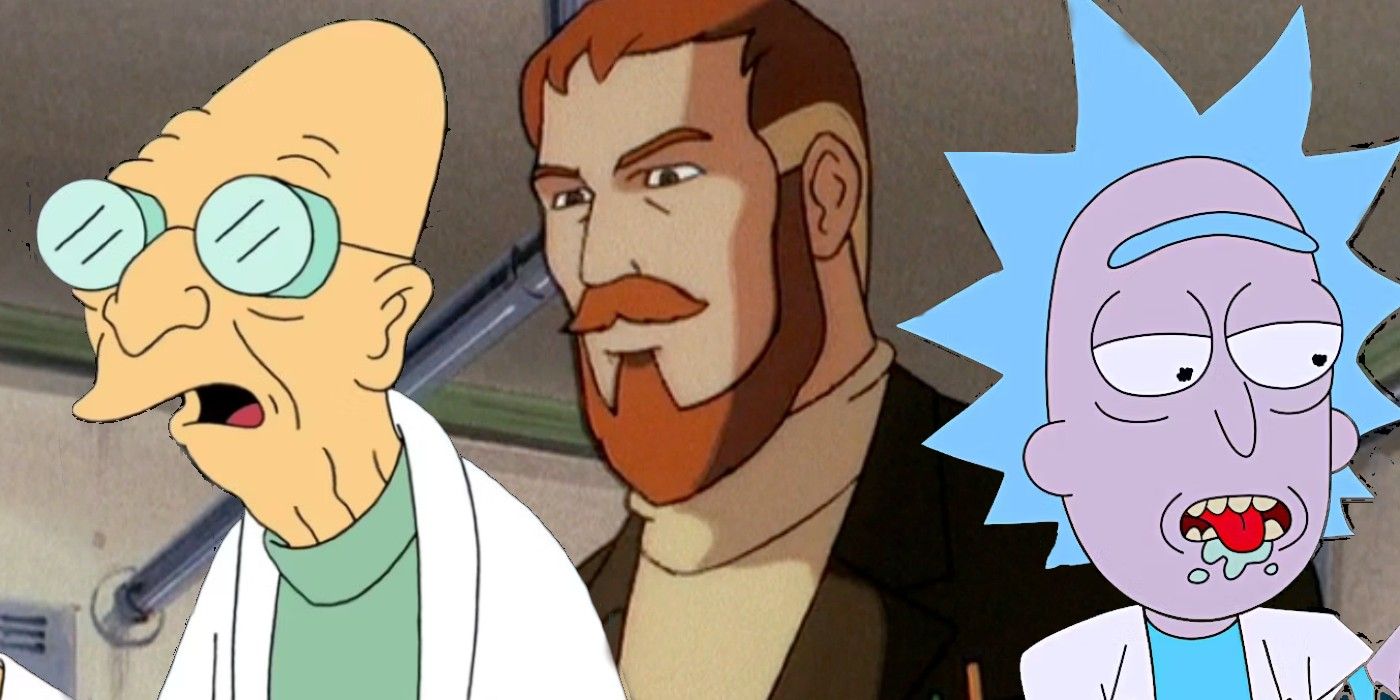This brightly colored, high-clarity cartoon screenshot features three animated characters. On the right, Rick from "Rick and Morty" is easily recognizable with his spiky light blue hair, bug-like large white eyes with small black irises, and a single unibrow. His skin tone is grayish, and he's depicted with his mouth open, revealing yellow teeth and a very red tongue with drool dribbling from his lip. He is dressed in his signature white lab coat and blue shirt. To the left, Professor Farnsworth from "Futurama" appears with his characteristically domed bald head, thick glasses, and a white lab coat over a green turtleneck sweater, making him look like an elderly scientist. Positioned centrally is a bearded man with reddish-brown hair and a contrastingly more naturalistic complexion. The background throughout the image is bright and clear, highlighting the vivid range of colors, including yellow, green, white, brown, beige, light blue, red, and purple. The entire scene is bathed in natural light, making the details of each character pop.